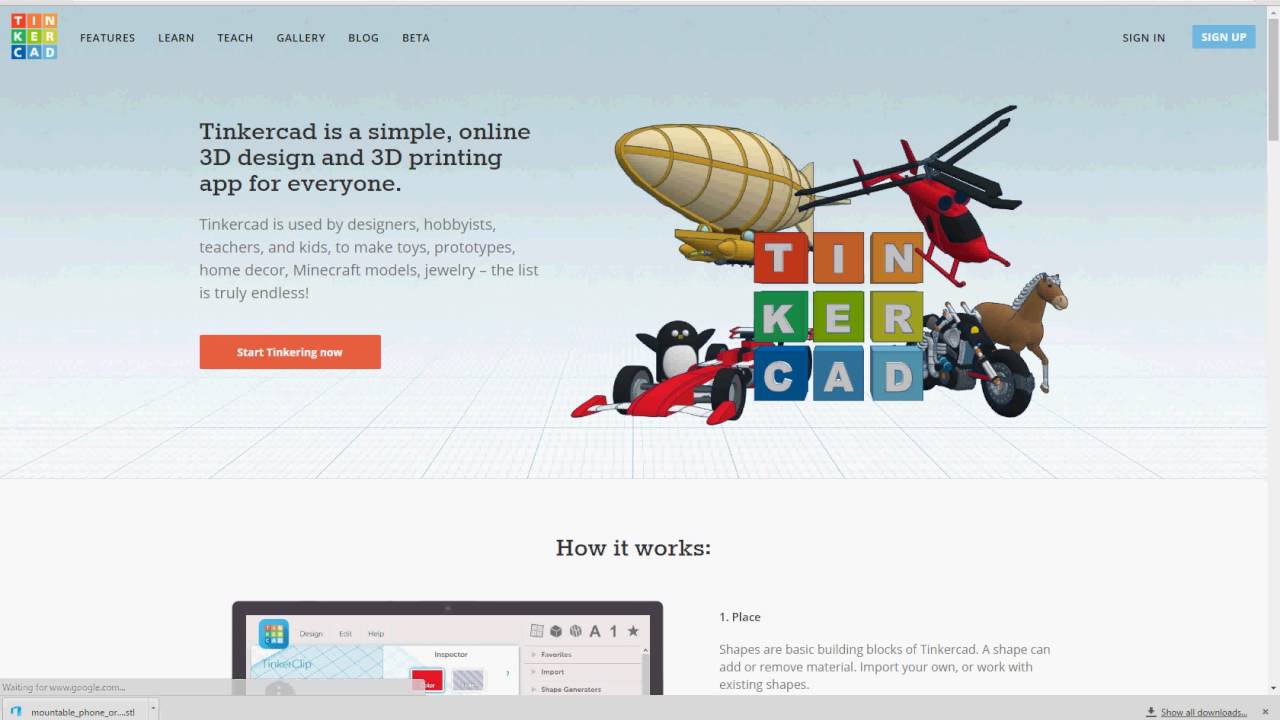This image is a detailed screenshot of the Tinkercad website, likely accessed at Tinkercad.com. The screenshot prominently features the Tinkercad logo in the upper left corner, comprised of nine boxes arranged in a 3x3 grid. Each box contains a letter, collectively spelling "Tinkercad," with each letter displayed in a distinct color.

Below the logo, the main body of the website showcases a variety of realistic yet cartoony clip art-style images, including a blimp, a helicopter, a horse, a motorcycle, an F1 car, and a penguin. These images add a lively and creative vibe to the webpage.

Central to the main content, another Tinkercad logo reiterates the site’s identity, flanked to the left by a description: "Tinkercad is a simple online 3D design and 3D printing app for everyone." A smaller paragraph follows, elaborating that Tinkercad is a versatile tool utilized by designers, hobbyists, teachers, and kids to create a wide array of items ranging from toys and prototypes to home decor, Minecraft models, and jewelry. The text emphasizes the limitless possibilities the app offers.

Concluding the introductory section, an inviting orange button labeled "Start Tinkering Now" entices users to begin their creative journey with Tinkercad.